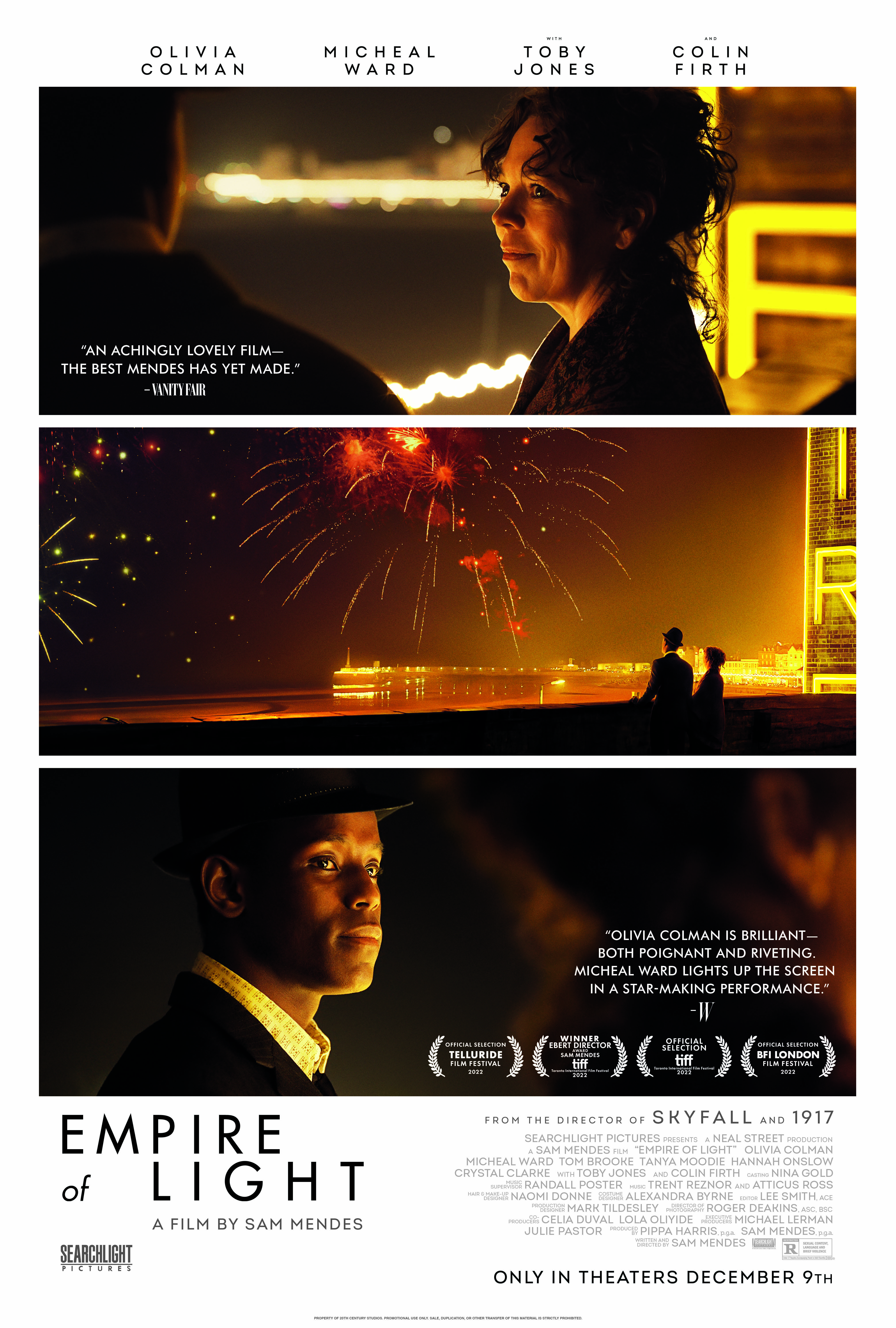The movie poster for "Empire of Light," a film by Sam Mendes, prominently features a series of three images that convey different scenes from the movie. The top of the poster lists the actors' names: Olivia Colman, Michael Ward, Toby Jones, and Colin Firth, with a small text excerpt from Vanity Fair praising the film as "an achingly lovely film the best Mendes has yet made." The first image at the top shows a woman on the right and a man on the left, with the woman gazing at the man. The middle section depicts the silhouettes of a man and woman standing by the water, watching fireworks illuminate the sky. The third image at the bottom shows a man and woman in a different pose, continuing their interaction. Below these images, the title of the movie is displayed: "Empire of Light," followed by the release information, "only in theaters December 9th," along with additional praise for the performances, "Olivia Colman is brilliant, both poignant and riveting; Michael Ward lights up the screen in a star-making performance." The poster is a rich tapestry of colors including yellow, white, light hues, reddish tones, brown, and black, creating a visually compelling and evocative preview of the film.